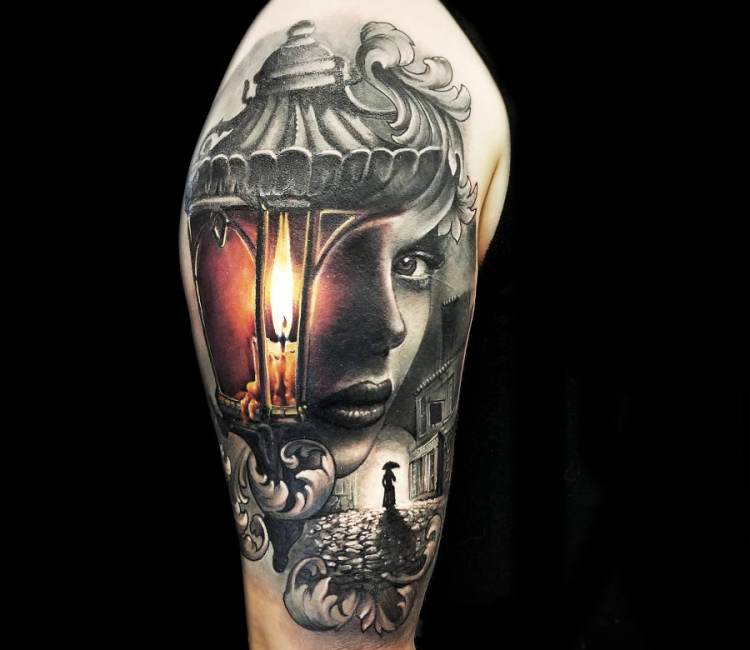This detailed image showcases a tattoo on a person's arm, against a black background. The tattoo, primarily in shades of grey, intricately depicts the side profile of a woman's face, capturing her one eye, nose, and mouth. Her hair morphs into the top of a structure resembling a temple or dome. Below this, a candle with a melting wax and a lit flame is positioned where her ear would be. The design continues with a cobblestone road that stretches into the distance, where the silhouette of a woman walking with an umbrella transitions from darkness to light. Surrounding this scene, additional structures and scroll-like designs are intricately shaded, adding depth and complexity. Leaves are scattered around the tattoo, and the person can be seen wearing a black shirt.